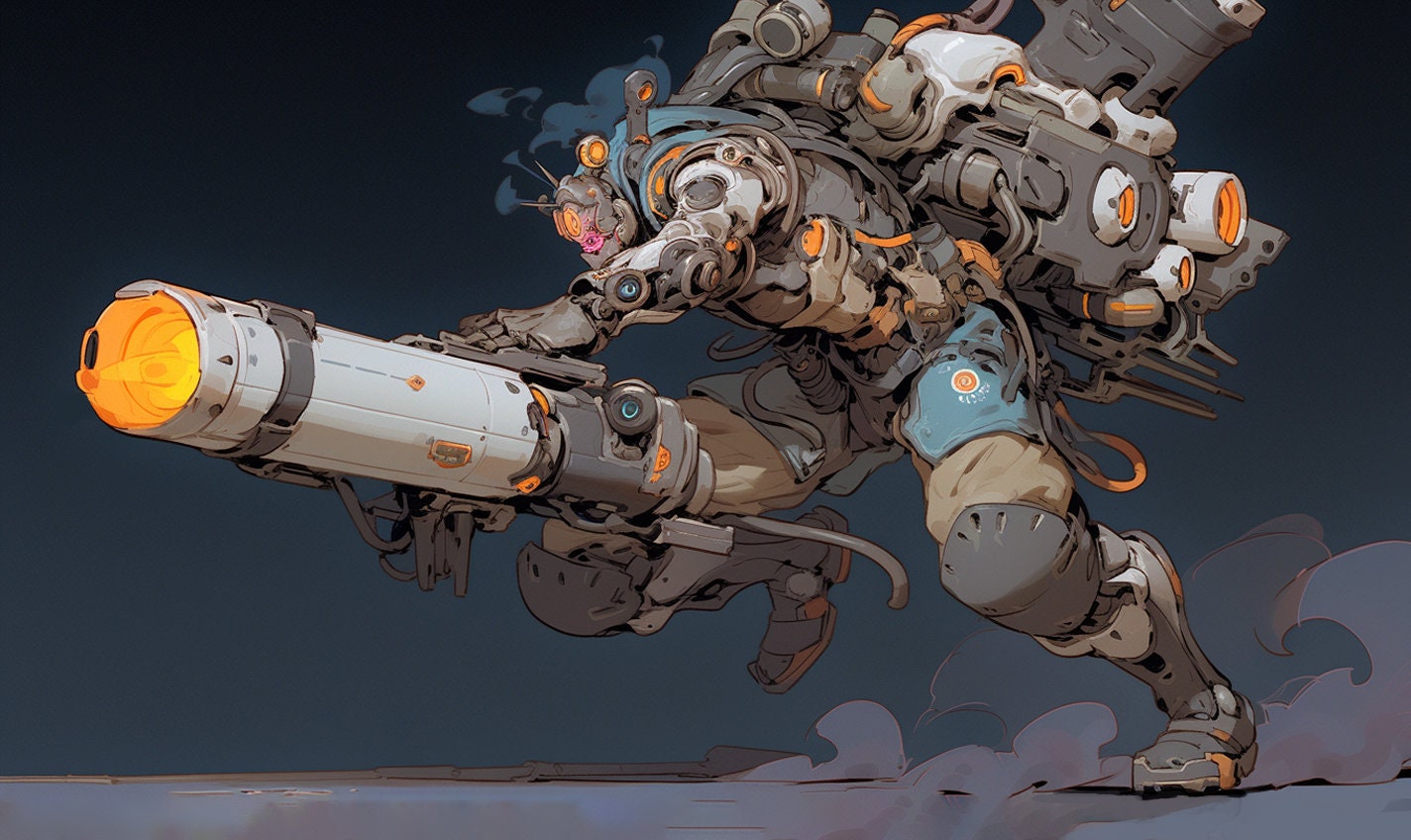This detailed illustration depicts an anime-style figure, possibly a mutant or alien, adorned in extensive military gear. The figure is heavily armored with tan fatigues, knee pads, and rugged combat boots. Despite its imposing and muscular build, it has an unusually small head, possibly due to the oversized body armor and intricate backpack it wears. This backpack is brimming with hoses, containers, and various pieces of machinery, suggesting it may be an energy source or weapons pack. Prominent among the figure’s gear is a massive weapon it's holding—a large, yellow-tipped device that resembles a powerful gun, be it a laser weapon or a fire-breather gun. This complex ensemble creates an imposing and futuristic warrior, ready for battle.